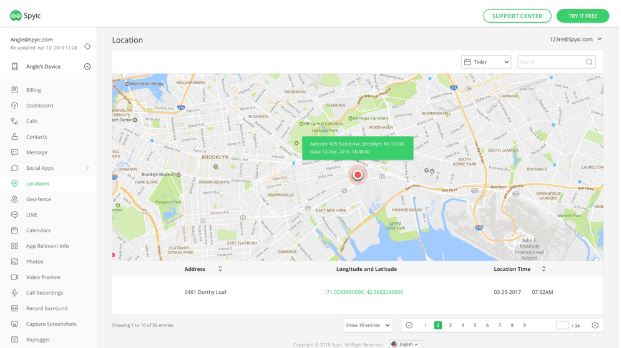This map, sourced from the website SPYIT, provides a detailed view of a section of New York City, focusing on the border area between Brooklyn and Queens. At the lower right of the image, John F. Kennedy International Airport is clearly marked. The Belt Parkway, a significant highway, is prominently featured, curving gracefully along the bottom and left side of the map.

Further details reveal the Van Wyck Expressway running vertically from north to south, intersecting with various other routes. A notable feature is a red dot centrally located on the map, likely indicating a specific point of interest or focal area. Directly above this red marker is a green box, though the text within it is too blurry to decipher.

Additionally, a green park is situated above the green box, providing some green space within the urban layout. Geographical demarcations indicate that the left portion of the map highlights the Brooklyn area, while the right portion outlines areas within Queens. The map seemingly extends upwards towards Manhattan, though it is not fully visible in this snippet.